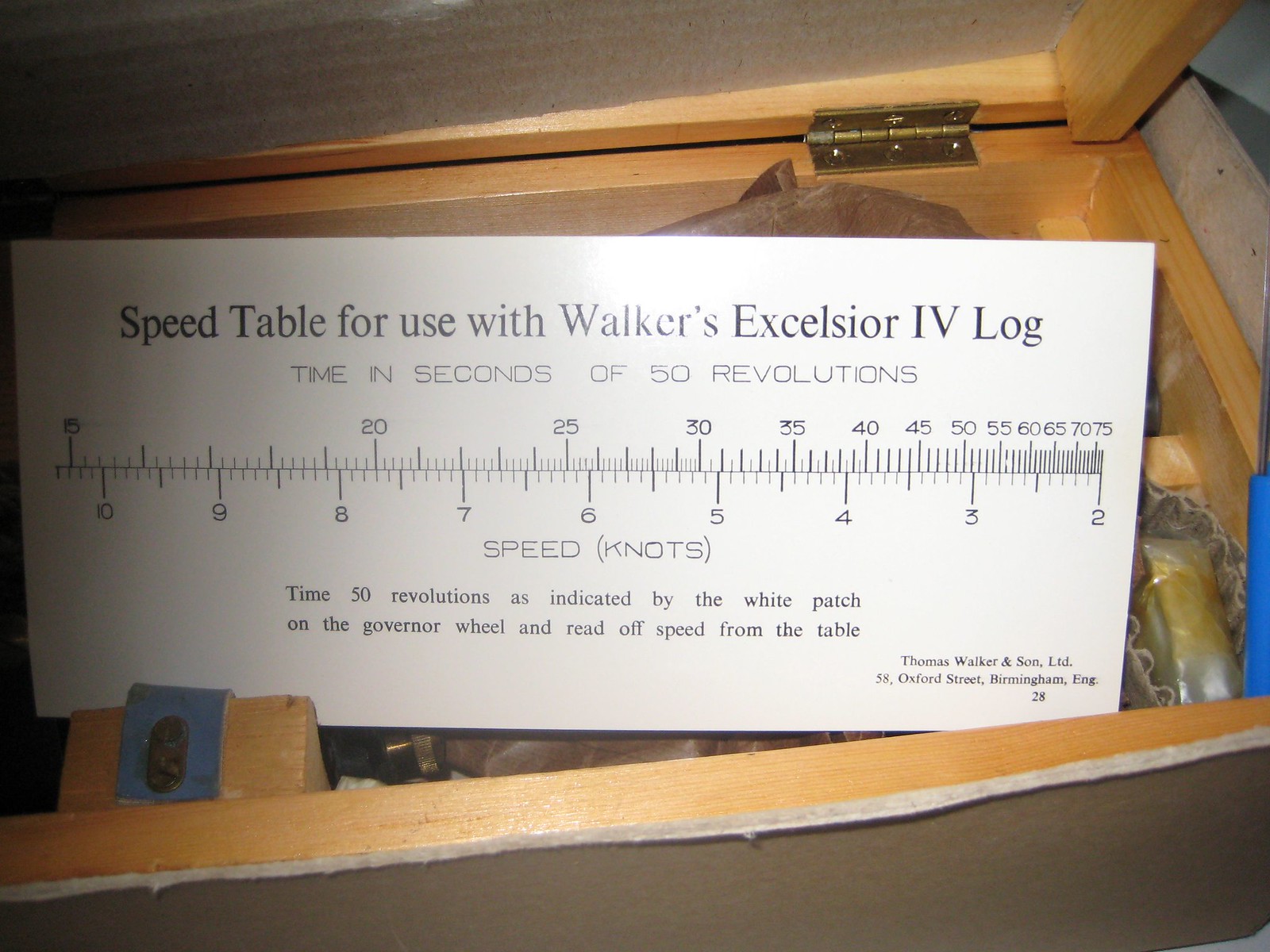The image depicts an open wooden chest containing a piece of paper detailed with nautical measurements and instructions. The paper prominently features a scale labeled "Speed table for use with Walker's Exerciser IV log." It provides a table indicating the "time in seconds for 50 revolutions," accompanied by a graduated number line where intervals become progressively closer towards the right-hand side. The top of the scale ranges from 15 to 75, while the bottom spectrum extends from 10 down to 2. The term "speed (knots)" is prominently labeled, indicating the nautical context of the document. At the bottom of the sheet, instructions read: "time 50 revolutions as indicated by the white patch on the governor wheel and readoff speed from the table," suggesting its use as a navigational aid. Given the chest’s sturdy and heavy wooden construction, it is likely that this setup is used aboard a boat rather than an aircraft.